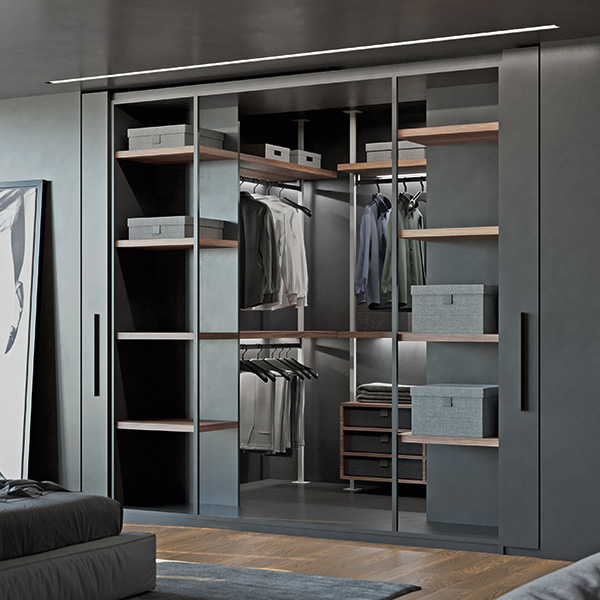This ultra-modern bedroom features a sleek, dark gray walk-in closet with an open design. The closet's steel-like color seamlessly integrates with the room's aesthetic. Inside, a sophisticated organization system includes built-in shelves adorned with elegant gray boxes, double-layered hanging sections with black hangers displaying white and dark shirts, and an integrated dresser at the bottom. A full-length body mirror leans stylishly against the left side of the closet. The room itself boasts a harmonious palette of various gray tones, complemented by a brown wooden floor partially covered by a gray rug. The edge of a bed with gray sheets is just visible, accentuating the cohesive decor. The closet, highlighted by its unique sliding doors, stands as a testament to modern design and functionality.